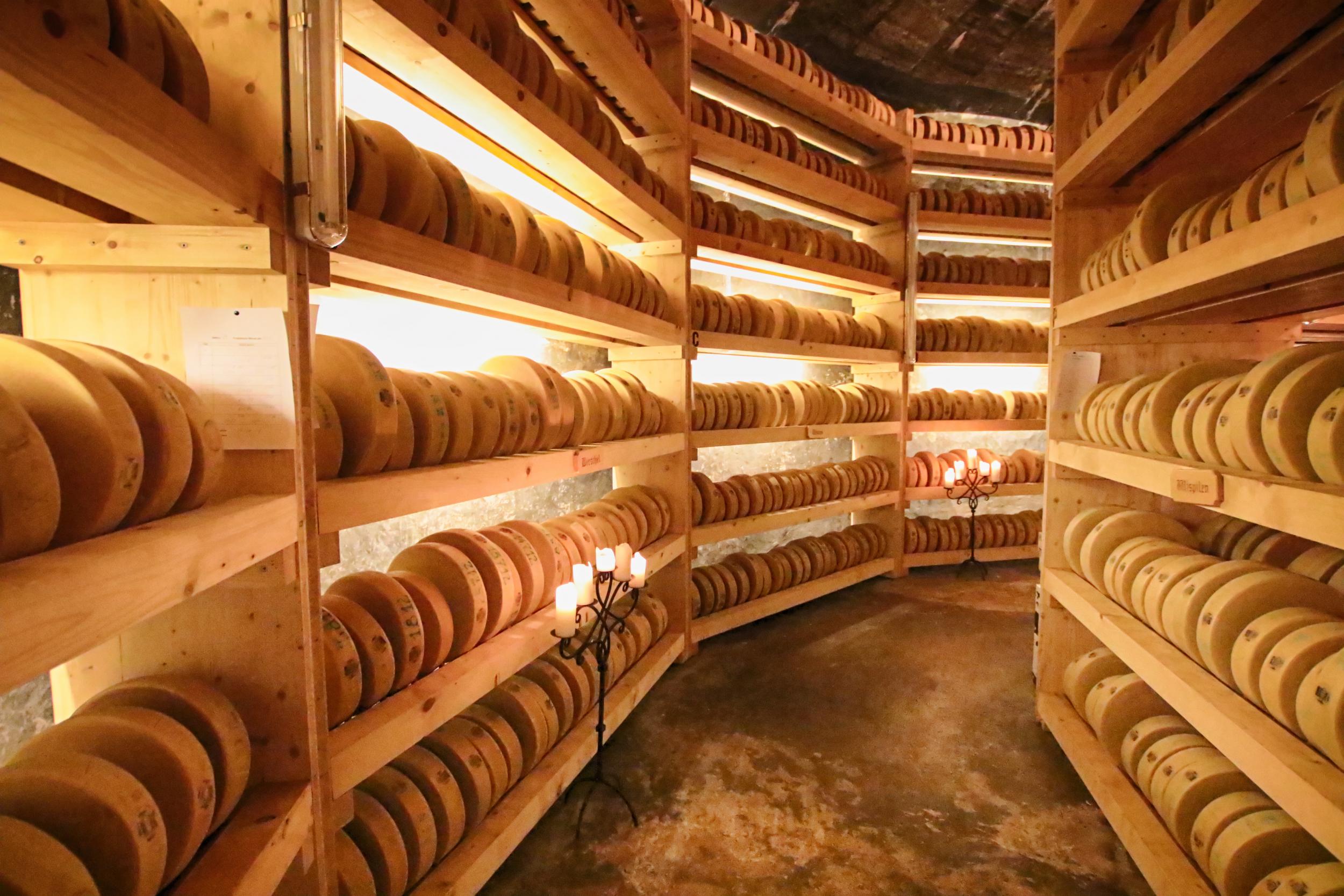The image captures a dimly lit, underground cheese storage room with wooden shelves lining both sides of a narrow walkway that curves sharply to the right. The room features a dark brown wooden ceiling and a brown marble floor, which gives it a slightly rustic appearance. The wooden shelves, which extend from floor to ceiling, are filled with numerous tan, disk-like wheels of cheese, each approximately as stacked horizontally and interspersed with occasional small dark spots or labels on their edges. There are seven shelves on each unit, visible as they stretch from the bottom to the top of the image, and disappearing as the walkway curves out of sight to the right. The cheese wheels are uniformly arranged, enhancing the room's orderly aesthetic. Adding to the room's dim lighting, stand-alone lights with multiple pronged tops and some candle-like features are positioned on the floor near the shelves, casting a warm, soft glow and emphasizing the underground, secluded feel of the storage area.